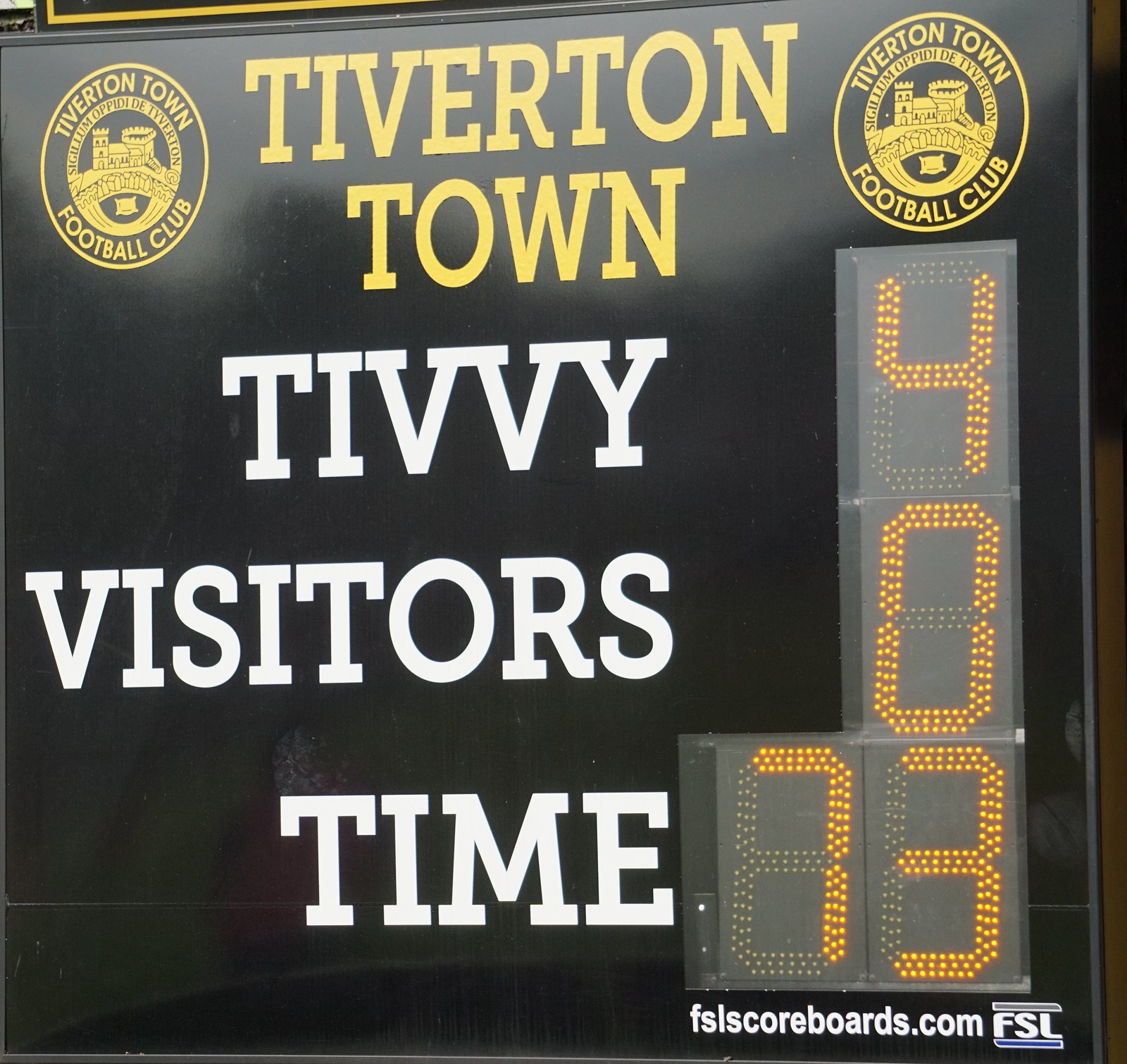The photograph depicts a scoreboard for a European soccer match, specifically the Tiverton Town Football Club. The scoreboard is black, adorned primarily with yellow and white text. At the top, in prominent yellow lettering, it reads "Tiverton Town," flanked by the club's logo on both sides—a gold circle featuring a castle with a bridge. Directly below, in white letters, it states "Tivy." The digital score beneath shows Tiverton Town leading with a score of 4, while the visitors have 0. The time is displayed as 73 minutes. At the bottom, it mentions "FSLScoreboards.com," indicating the scoreboard provider.